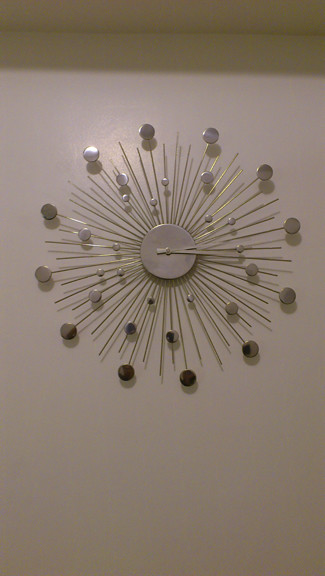The image features a rectangular frame, approximately two and a half times taller than it is wide, set against a background of a wall that appears off-white or light brown due to the dim interior lighting, giving it a slight grayish pink hue. About 5% down from the top, the wall intersects with the ceiling, which shares the same shaded color. Centrally mounted on this wall is an abstract, difficult-to-read clock with a starburst design. The clock has a core silver circular base with two silver hands indicating a time close to 3:16 or 3:17. Radiating out from this central circle are about 20 to 30 brass rods of varying lengths, arranged like a sunburst. Some of these rods feature silver discs of different sizes, resembling the size of quarters, at their ends. Shadows from the rods against the wall and a white highlight, possibly from the camera flash, add depth to the image.